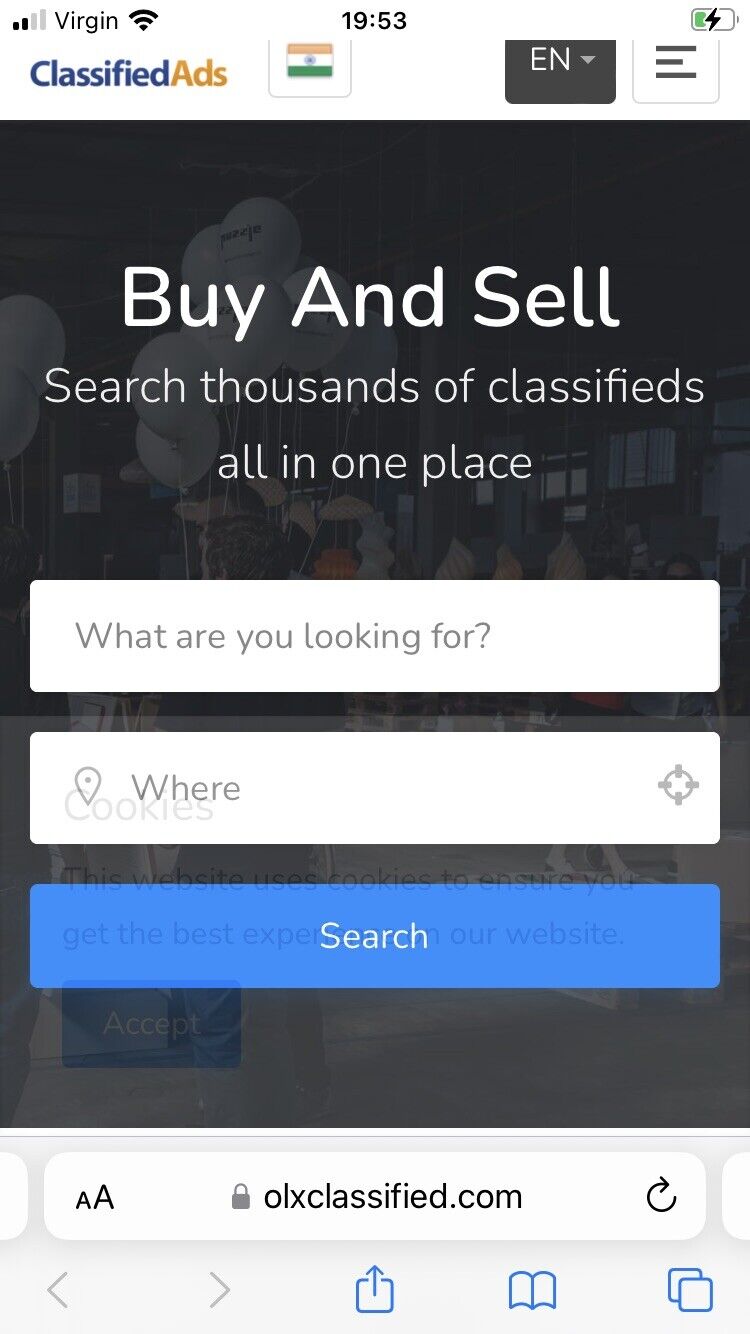A mobile screenshot displays a classified ads website or app. Atop the screen, the device's status bar shows the cell signal strength, Wi-Fi connection, and the carrier, Virgin Mobile. It's 19:53, and the battery icon on the right indicates that the phone is charging. Beneath the status bar, the app's header features the words "Classified Ads" with "Classified" in blue and "Ads" in orange, accompanied by a flag icon and an English language setting menu on the right side.

Underneath the header, against a black background, there appears to be an image of a marketplace or fair with various shops or booths. Balloons are visible at the top, and people can be seen in the background. The app's tagline, "Buy and sell. Search thousands of classified ads all in one place," is prominently displayed.

Further down, there's a search bar prompting "What are you looking for?" followed by fields to specify location and a search button for users to initiate their query.